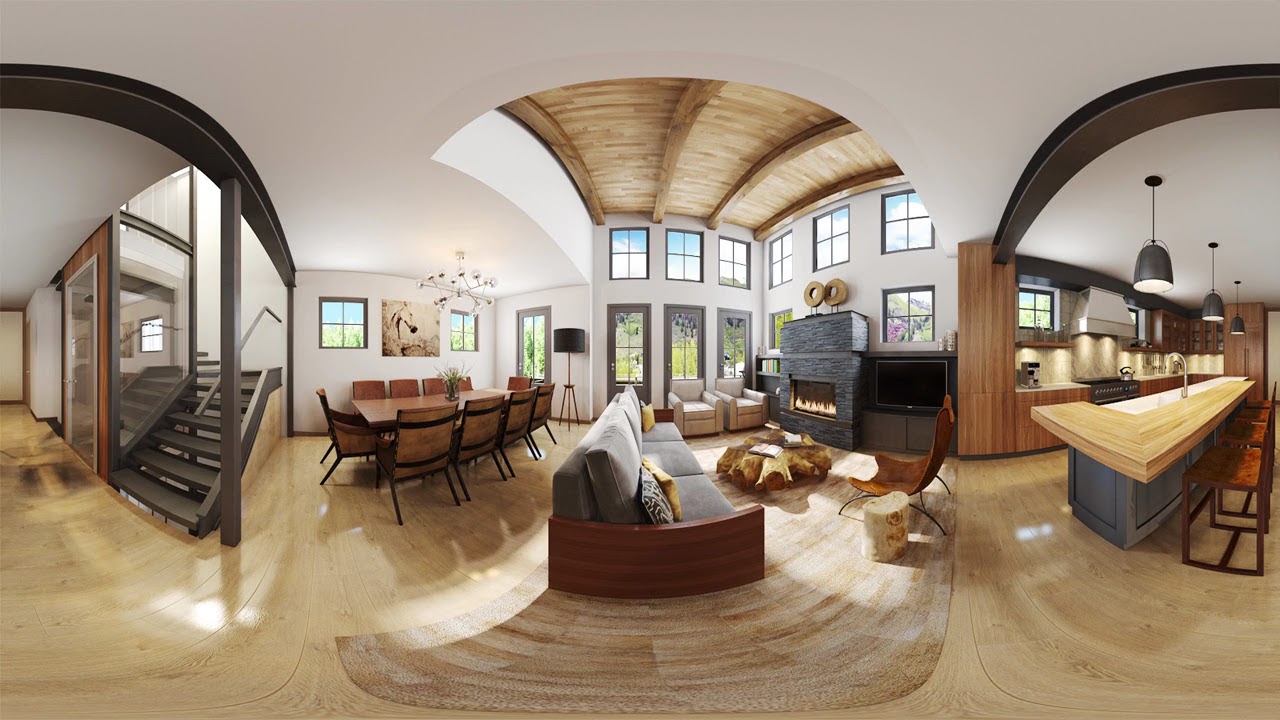This panoramic indoor image showcases a spacious and well-lit part of a house featuring a seamless blend of living, dining, and kitchen areas. At the center is the living room with a grey couch, a grey fireplace ablaze, and a television set, all framed by multiple high windows and wooden floors. Behind the living area, a dining table with ten chairs is situated, accented by a painting of a horse on the white walls and a chandelier hanging overhead. To the right, the modern and upscale kitchen boasts wood cabinets, a wood countertop, grey cabinetry underneath, hanging lights, and a coffee maker on the countertop. On the extreme right is a bar area with seating, blending seamlessly into the kitchen. To the left, a wooden stairway enclosed by glass panels leads to the upper part of the house, and sliding glass doors open to other areas of the home that are not in view. The entire scene is unified by its wooden elements, extending from the floor to the ceiling, contributing to the warm and cohesive aesthetic of the space.